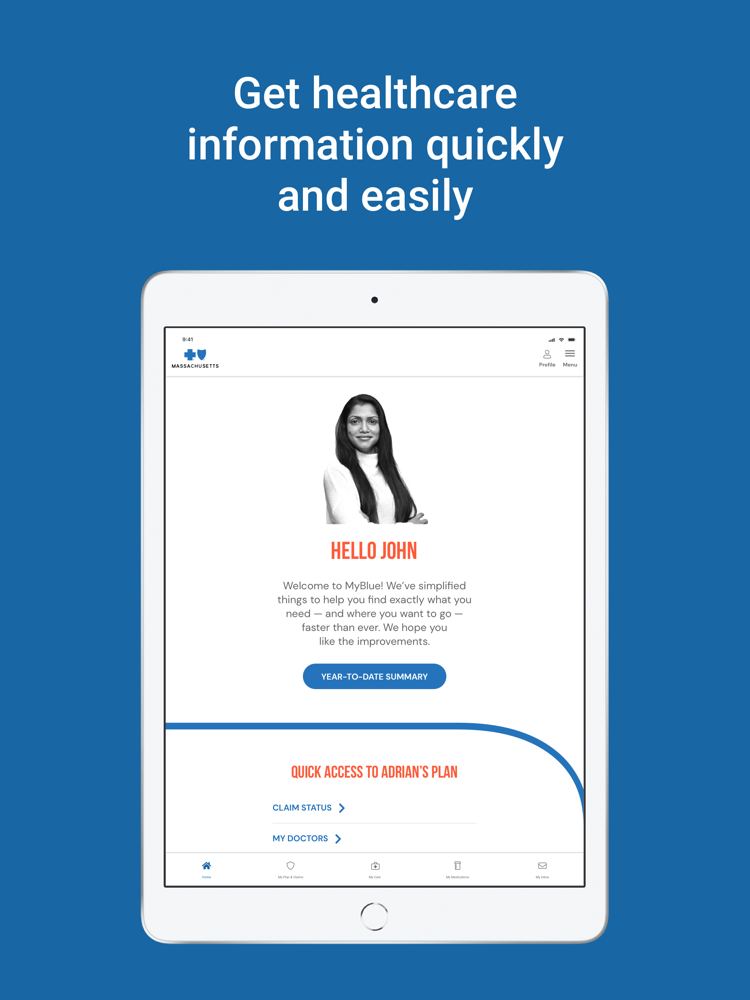In the image, a person with long hair and wearing a white shirt is gazing forward at an iPad positioned at the top of a shelf. The iPad's screen displays the Blue Cross Blue Shield logo prominently at the top, along with a greeting saying "Hello John, welcome to My Blue." The interface aims to simplify healthcare information, offering quick access to essential features like Adrian's plan, claim status, and doctor's information. 

The background of the image is a calming blue, enhancing the sense of ease and accessibility. Various icons are visible on the screen—five in total—each representing different options available to the user. A navigational bar includes a hamburger menu icon, indicating additional options. In red text, "Quick Access to Adrian's Plan" is highlighted, while other features like "Claim Status" and "My Doctors" are presented in blue text, accompanied by a right-pointing chevron indicating more details can be found by tapping these options. The overall message conveys that the improvements made will help users find exactly what they need quickly and efficiently.